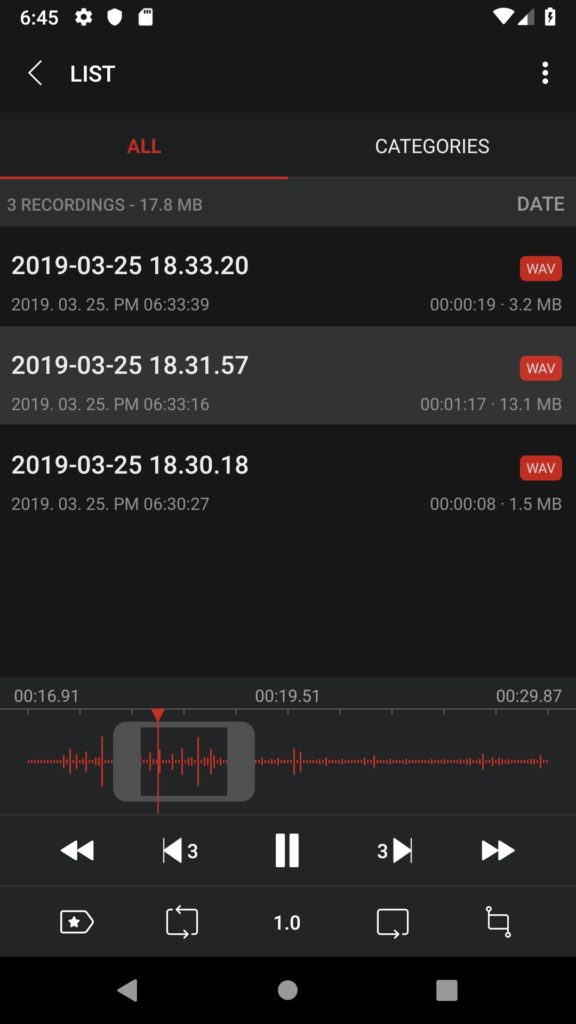Screenshot of a mobile recording app interface:

At the very top of the screenshot is the phone's status bar, displaying the time as 6:45 (either AM or PM) on the top left. Adjacent to the time are three icons: a cogwheel, a shield, and a page icon. On the top right, there are icons for Wi-Fi signal, LTE signal, and battery percentage.

The main body of the app interface begins below the status bar. In the top left corner, the word "List" is displayed in white, accompanied by a left-pointing arrow. On the top right are three vertical dots, indicating additional options. Below this toolbar, there are two tabs labeled "All" and "Categories." The "All" tab is selected, highlighted in red with a red underline.

The main content area of the screen shows a list of three recordings. Each recording entry displays its date and time on the left side, and on the right side, it shows details such as format, length, and file size. The first recording is listed as 17.8 megabytes.

At the bottom of the screenshot is a waveform display in red, representing the audio waves of the recording. A gray box encompasses a portion of the waveform, allowing the user to move this section back and forth for precise navigation through the audio.

Finally, the playback controls are positioned at the very bottom of the screen. They include buttons for fast rewind, rewind, pause (centered), fast forward, and fast fast forward.